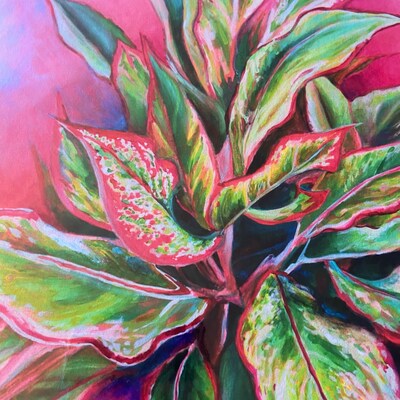This is a very detailed, close-up watercolor painting of a plant with large, vibrant leaves. The painting is a riot of colors dominated by pinks, greens, and blues, creating an almost explosive effect. The leaves are a complex mix of dark to light greens, pastel reds, yellows, and shades of pink. The plant's stem is primarily pink with hints of black. The veining on the leaves is a purplish-pink, adding intricate details to the artwork. The background is a pink haze that fades into light blue towards the top left, enhancing the plant's vivid colors. There are about 10 to 20 leaves forming a triangular shape, with the middle top leaves facing upwards and the bottom leaves splaying outwards. Blue-green tones and royal blue shadows add depth and dimension to the composition, making it a visually dynamic piece.